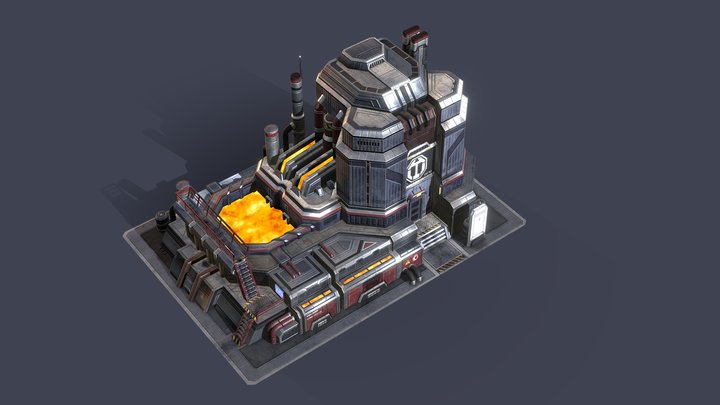The image depicts a detailed model of a factory-like building set against a straight gray background, creating a stark and industrial appearance. The factory model features various ladders and compartments, with a prominent entrance gate situated on its right side. Central to the model is an area where a yellowish liquid, resembling yellow lava, is pouring out in two streams and being stored openly in the middle section of the building. The structure is primarily gray with accents of white and yellow, contributing to its mechanical and somewhat futuristic look, suggestive of a cyberpunk aesthetic. The shadow of the building is also visible, adding depth to the image, which is angled in a way that provides a top-down perspective on the factory’s layout.